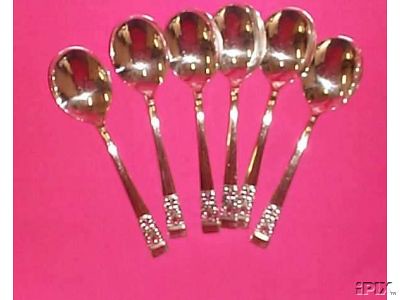The photograph captures six short golden spoons meticulously arranged side by side on a bright pink background. Each spoon lies horizontally with the rounded, polished bowl facing the top of the image and the handles pointing downward. The handles, which feature a delicate, ornate design resembling silver or diamond encrustment on their ends, add a touch of elegance to the otherwise solid gold spoons. Despite the low resolution and slight blurriness of the image, the intricate details and brilliant shine of the golden spoons stand out. In the lower right corner, a partially visible watermark, potentially reading IPLTM or IPDC, subtly asserts its presence.